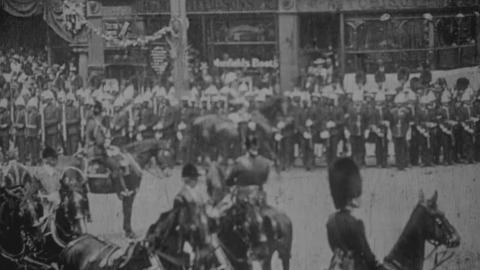This black-and-white photograph, although of poor quality, captures a significant historical moment depicting a line of troops standing in front of a store. The soldiers, all dressed in dark uniforms, are uniformly equipped with hats or helmets, adding to the disciplined appearance of the scene. In the foreground, closer to the camera, several individuals are mounted on horses, adding a dynamic element to the composition. Among the soldiers, one stands out distinctly; he is wearing a notably tall black fur hat, which adds a unique focal point to the image. Despite the graininess and lack of clarity, the photograph exudes a sense of historical gravity and disciplined military presence.